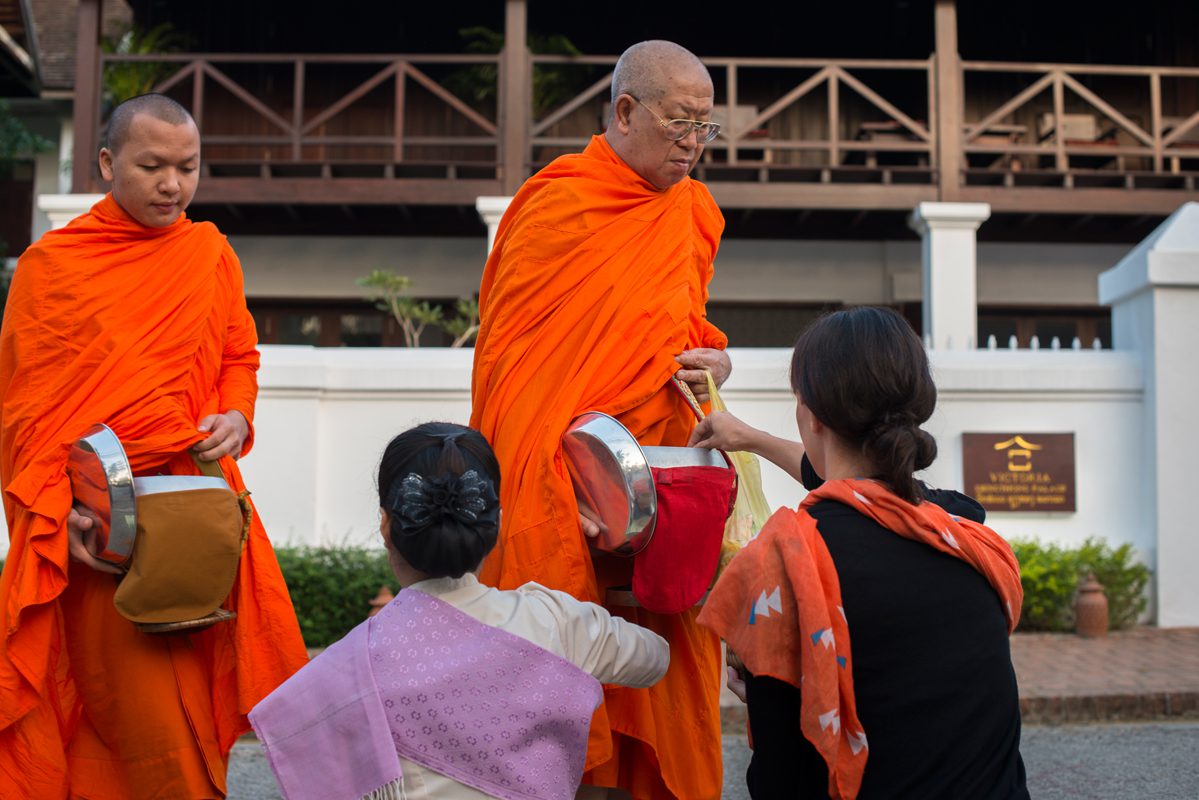In the photograph, taken outdoors in front of a building, a serene scene unfolds against a backdrop of a white wall lined with low hedges. The setting features a brick sidewalk elevated from the street, leading up to a wooden platform adorned with tables, chairs, and planters filled with vibrant potted plants, suggesting an open porch. In the foreground, on the street, stand two Buddhist monks in orange robes, one with very short hair and the other bald with gold metal-framed glasses. The monk with glasses is holding a red bag and a metal donation platter. Both monks have satchels draped around their waists.

Approaching the monks are two women, their backs turned to the camera. One woman is dressed in black with an orange scarf wrapped around her, while the other wears a white dress with a thick purple scarf draped over her shoulder. The women, each with their hair pulled back into buns, appear to be kneeling before the monks. The woman in black is actively placing something into the satchel of the monk on the right, indicating that they are giving donations. The overall ambiance suggests a ritualistic or religious donation ceremony taking place in a peaceful, perhaps oriental religious context.